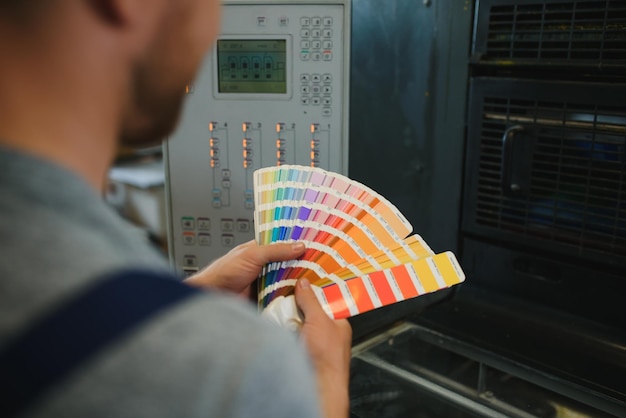In this photorealistic image, a bearded man with a gray shirt and a blue strap visible over one shoulder holds a large fan of color paint samples in his hands. The samples, fanning out to display a spectrum from tan to green, purple, pink, red, orange, and yellow, are the main focus as they vividly contrast with the blurred figure. The man stands in front of a complex machine that likely mixes or shakes paint, characterized by a gray monitor with numerous colored, lit buttons and a screen displaying cryptic rectangular images with black squares. To the side, a black grilled panel with a handle adds to the industrial setting. The backdrop includes a gray wall and a black door handle, contributing to the sense of a controlled, mechanical environment designed for precise operations.